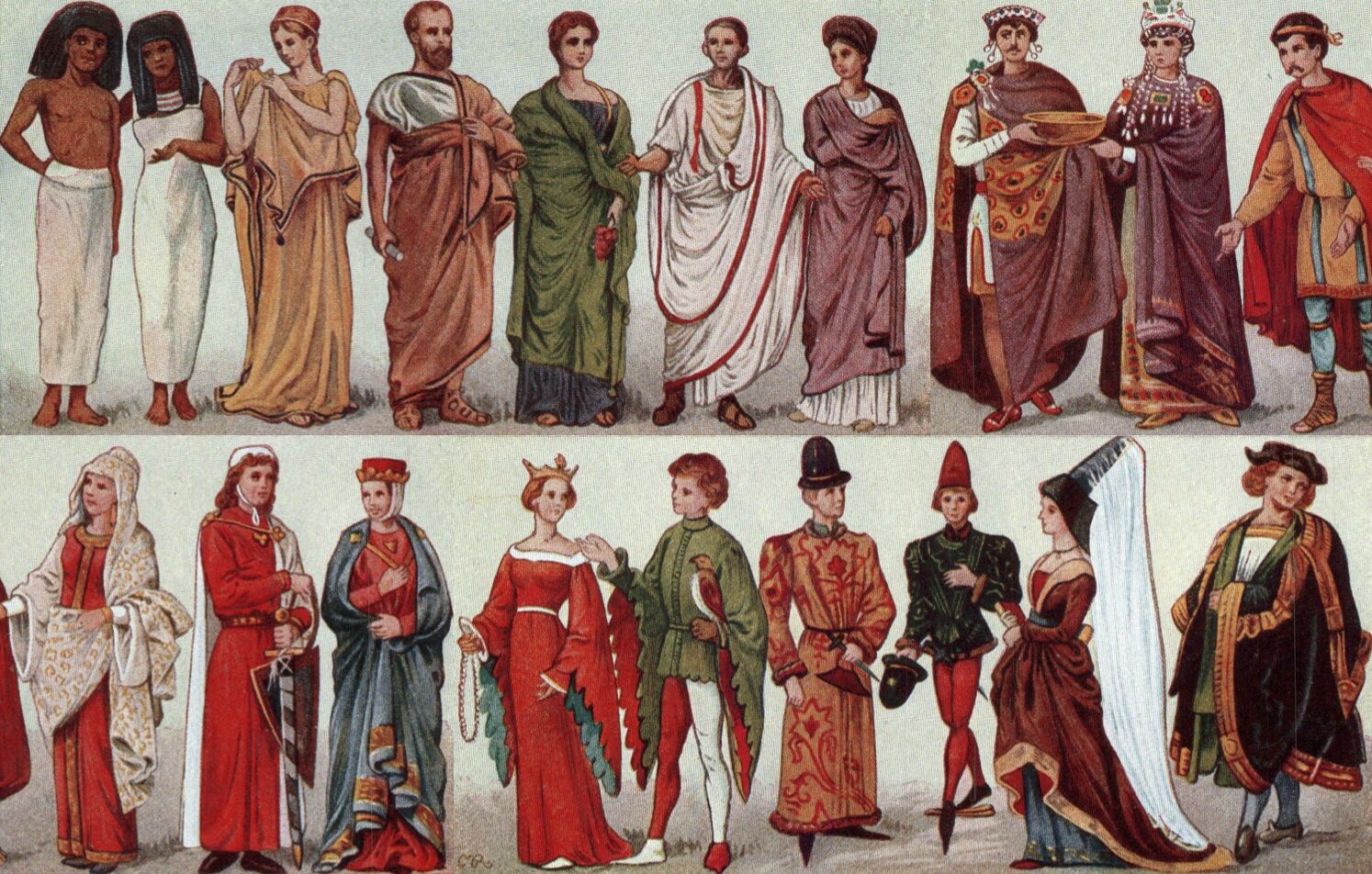The image consists of two horizontally aligned rectangular illustrations stacked one above the other. Each image features a group of people dressed in intricately designed, historically-inspired attire, resembling a progression of eras from ancient to more recent times. 

In the upper illustration, there are 11 individuals, a blend of men and women, wearing robes and gowns in various colors such as brown, red, and some green. Among them are two dark-skinned figures on the far left— a shirtless man in white pants and a woman in a white jumper. The rest of the figures are adorned with crowns and an abundance of beads over their robes. Notably, a central figure resembles a Roman or Greek figure, dressed in a white robe with red trim, possibly evoking the image of Caesar. 

The lower illustration showcases 10 people, characterized by more pronounced red garments. One standout figure is a woman in a dark red gown with gold trim, wearing a feathery hat with a long veil. Another notable figure on the far right, dressed in an elaborate gown, resembles historical figures like Christopher Columbus. The illustrations collectively convey a transition through historical eras, from ancient Egyptian to a Renaissance or possibly Tudor period, reminiscent of the fashion and royalty associated with figures like Henry VIII or the characters in "Romeo and Juliet."